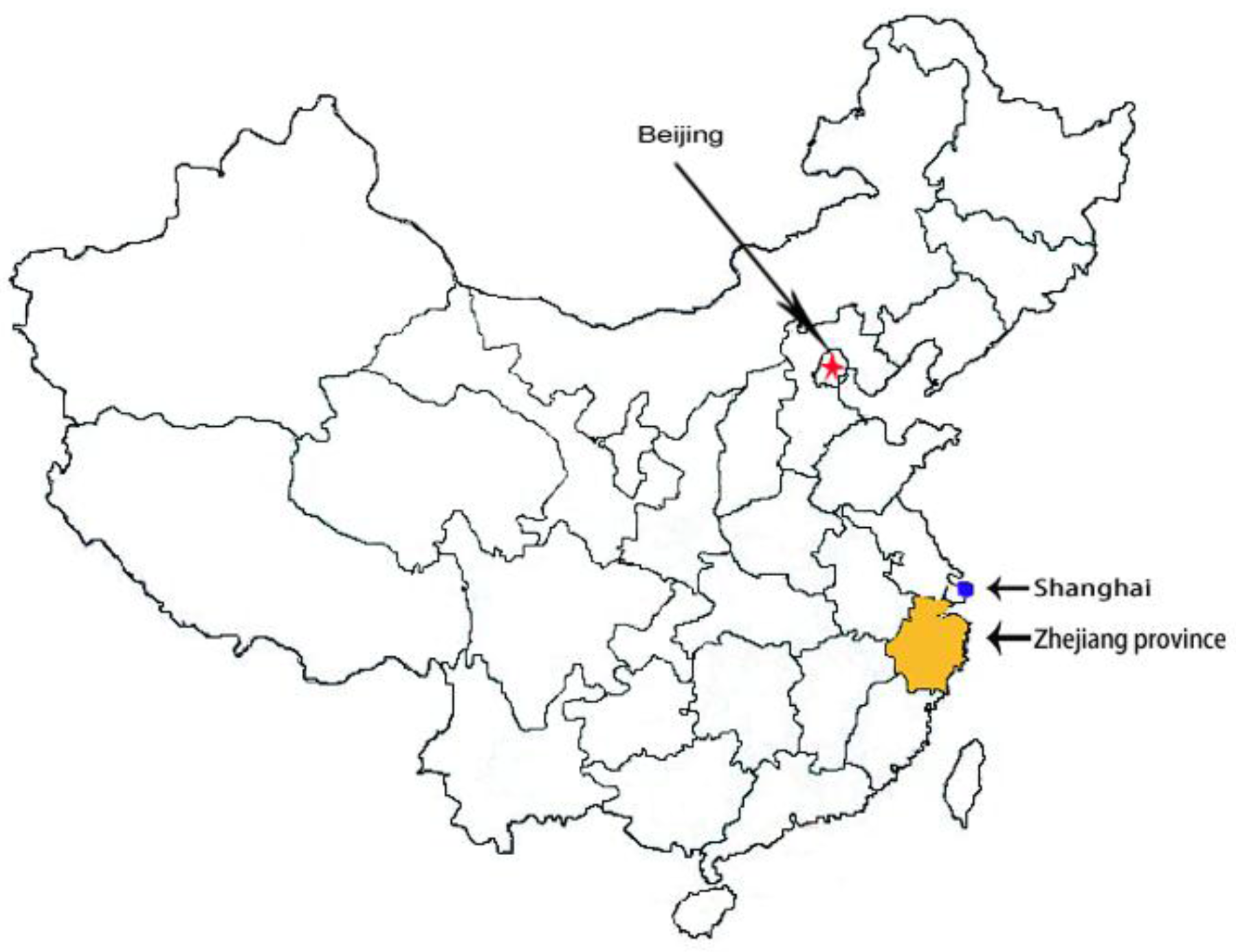This image features a simplified map of China, outlined in black on a white background with provincial boundaries clearly marked. The most prominent details are three labeled locations. To the upper right-center, a red star denotes Beijing, indicated by a diagonal black arrow originating from the upper left with the label "Beijing." In the middle-right section, a blue dot marks Shanghai, also highlighted by an arrow pointing rightwards with the adjoining label "Shanghai." Below Shanghai, the Zhejiang province is highlighted in yellow, with an identifying arrow and label "Zhejiang province" to the right. The map's design is minimalistic with these three annotations being the only highlighted and labeled elements.